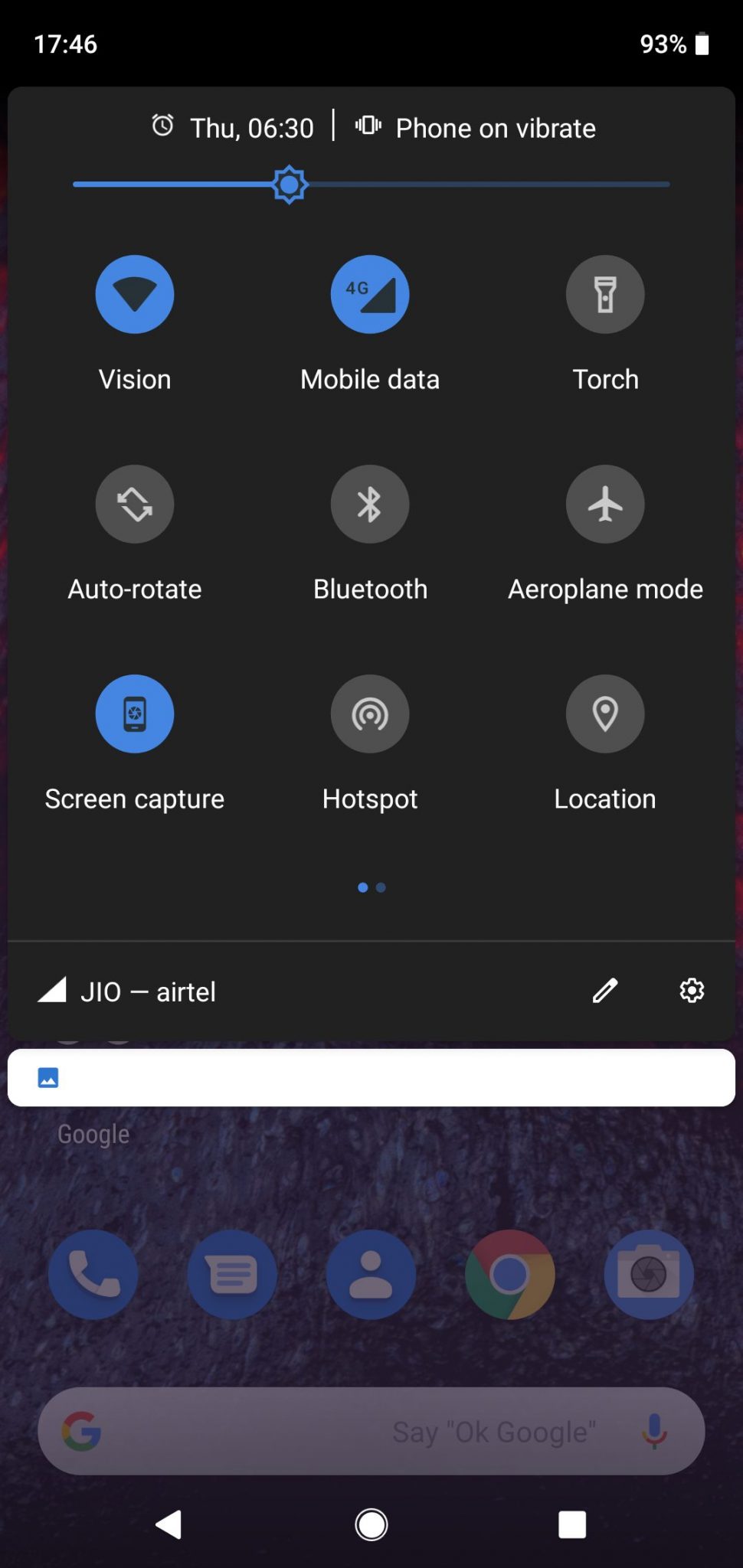This image is a screenshot taken from a smartphone in portrait mode. The top and bottom sections of the screen are dark black while the middle part is a regular black. In the top left corner, the time reads 17:46, and in the top right corner, the battery shows a 93% charge. Directly beneath this, on a very dark gray background, there are several status icons: an alarm clock, indicating an alarm set for Thursday at 6:30, and a phone on vibrate.

The screen's brightness level is approximately 40%. The following row features three icons: a blue-lit indicator for mobile data (showing 4G), and a flashlight icon labeled "Torch" which is not lit up. Below this, there are icons for Auto Rotate, Bluetooth, and Airplane Mode – none of which are activated. The next row contains icons for Screen Capture, Hotspot, and Location. The Screen Capture icon is lit up, while Hotspot and Location are not active.

At the bottom of this section, two small blue dots indicate the current page within a multi-page interface. Below this, there are carrier names "Jio" and "Airtel" separated by a slash. The lower portion of the screen features a large search bar, followed by several Google app icons.